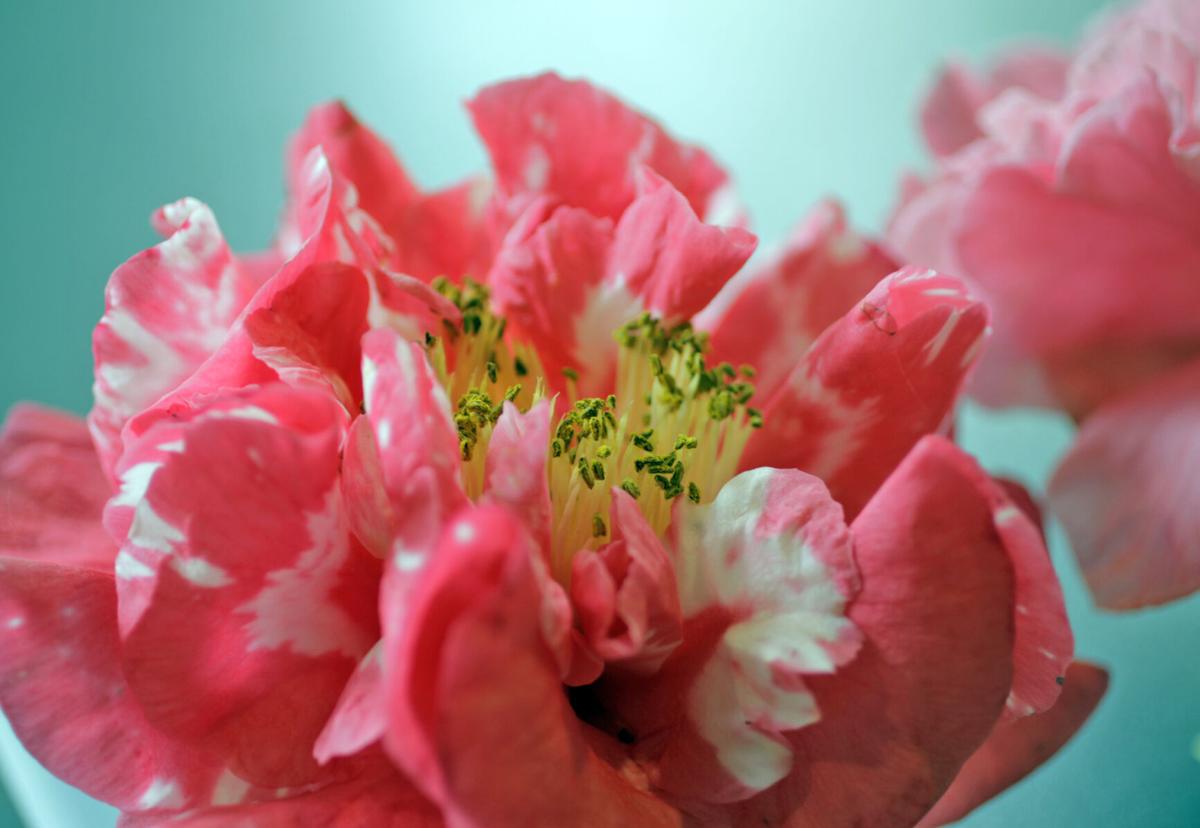This image is a close-up of a predominately pink flower with white accents on its petals, occupying about 90% of the frame's height and extending from the left edge, slightly cut off, to about 95% of the right. The petals sweep gracefully upwards and then curve back down, creating an open bloom. At the flower’s center, celery-green stems topped with tiny hunter green balls, or buds, create a striking contrast. The setting features a blurred backdrop in shades of teal and light teal, which enhance the flower's vibrant colors. Slightly out of focus and positioned on the upper right side of the image, another similar flower appears, showing about 20-30% of its structure. The entire composition is angled downwards, capturing the main flower in significant detail while leaving the second flower partially visible in the background.